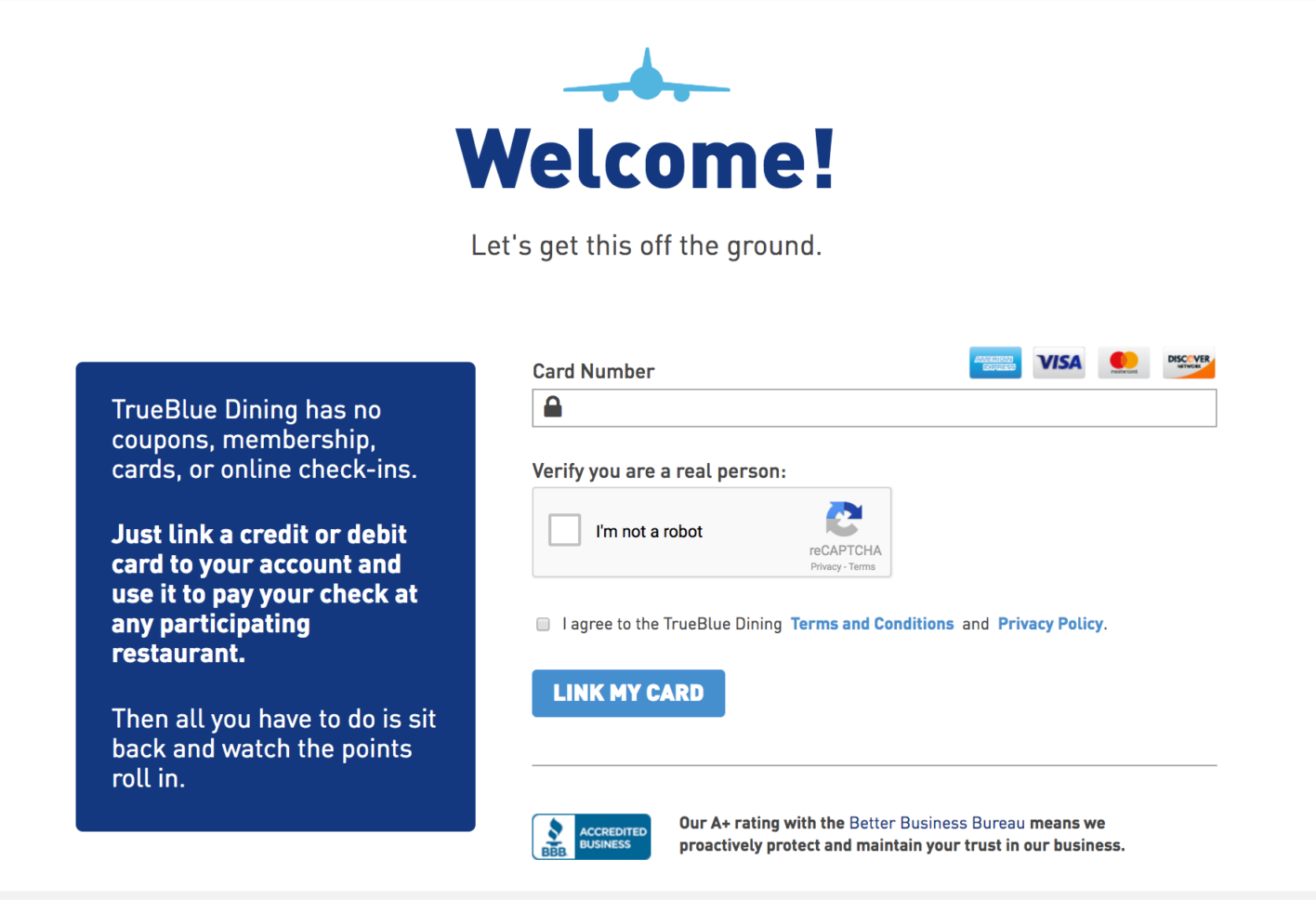In the image, we see a screenshot of a website's landing page. At the top of the page, "Welcome!" is displayed in dark blue text, accompanied by an airplane logo in light blue just above it. Directly below the welcome message, another line of text reads, "Let's get this off the ground."

On the left side of the screen, there's a blue square divided into three sections, each containing white text. The top section states, "True Blue Dining has no coupons, membership cards, or online check-ins." The middle section explains, "Just link a credit or debit card to your account and use it to pay the check at any participating restaurant." The bottom section summarizes, "Then all you have to do is sit back and watch the points roll in."

To the right of the blue square, a section for entering a card number is displayed, featuring a rectangular input field. Above this field, there are four logos of popular credit cards. Below the input field, users are prompted to "Verify you are a real person," with a checkbox labeled "I'm not a robot." Further down, there's another checkbox labeled "I agree to the True Blue Dining terms and conditions and privacy policy."

At the bottom of this section, a blue rectangular button with white text says "Link My Card." Just below this button, a thin horizontal line stretches across the screen. Below the line, a label has a dual background: white on the left and blue on the right. On the right side of this label, a message reads, "Our A+ rating with the Better Business Bureau means we proactively protect and maintain your trust in our business."